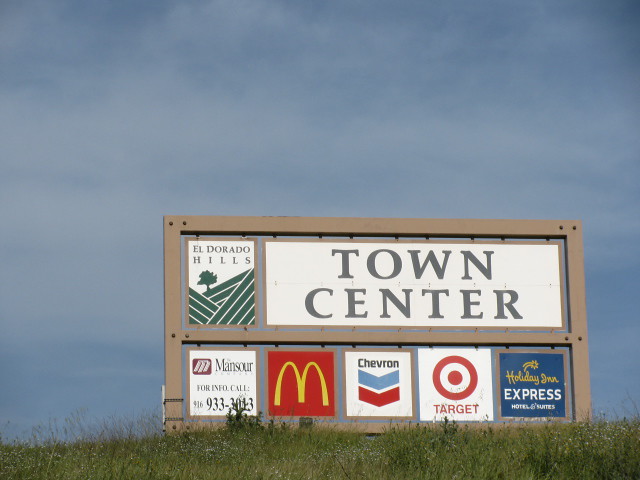The photograph is a wide-angled shot capturing an elaborate series of billboards situated along a highway. At the forefront, a verdant grassy field stretches across the bottom of the frame, while the top is dominated by an overcast blue sky, indicating daytime.

At the center of the image stands a wooden-framed billboard, divided into two main sections. The upper portion prominently features "Town Center" and an additional rectangular section with "El Dorado Hills" inscribed. Below, a series of square advertisements display various establishments in the shopping center or accessible from this highway exit. These include "Monsoor" with a note for more information, McDonald's, Chevron, Target, and Holiday Inn Express Hotel & Suites.

Unlike typical highway exit signs, this billboard exudes an air of sophistication and deliberate effort, designed to convey an upscale and appealing destination.